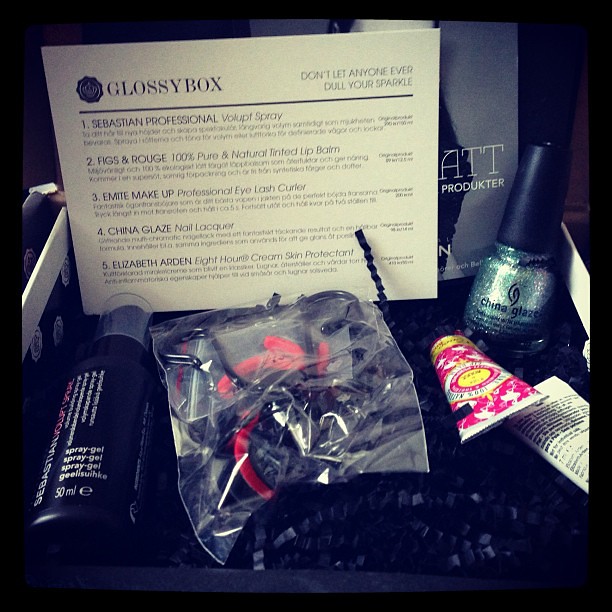The image showcases a promotional display for a beauty subscription box, "Glossy Box," with the slogan "Don't let anyone ever dull your sparkle" prominently displayed at the top. The featured products include:

1. **Sebastian Professional Volupt Spray** - A black bottle of volumizing spray.
2. **Figs & Rouge 100% Pure and Natural Tinted Lip Balm** - A lip balm positioned on the right side, identifiable by its pink packaging.
3. **Emmit Makeup Professional Eyelash Curler** - A high-quality eyelash curler.
4. **China Glaze Nail Lacquer** - A nail polish in a green bottle placed on the right side.
5. **Elizabeth Arden 8-Hour Cream Skin Protectant** - A white tube of skin protectant on the right.

The detailed card listing and describing these products is placed at the top of the image, while the items themselves are neatly arranged at the bottom. The setting appears to be indoors, suggesting this layout could serve as an advertisement or promotional image for the Glossy Box beauty subscription service. The colors present in the image include black, white, off-white, gray, green, pink, purple, red, and yellow, adding vibrancy and appeal to the presentation.